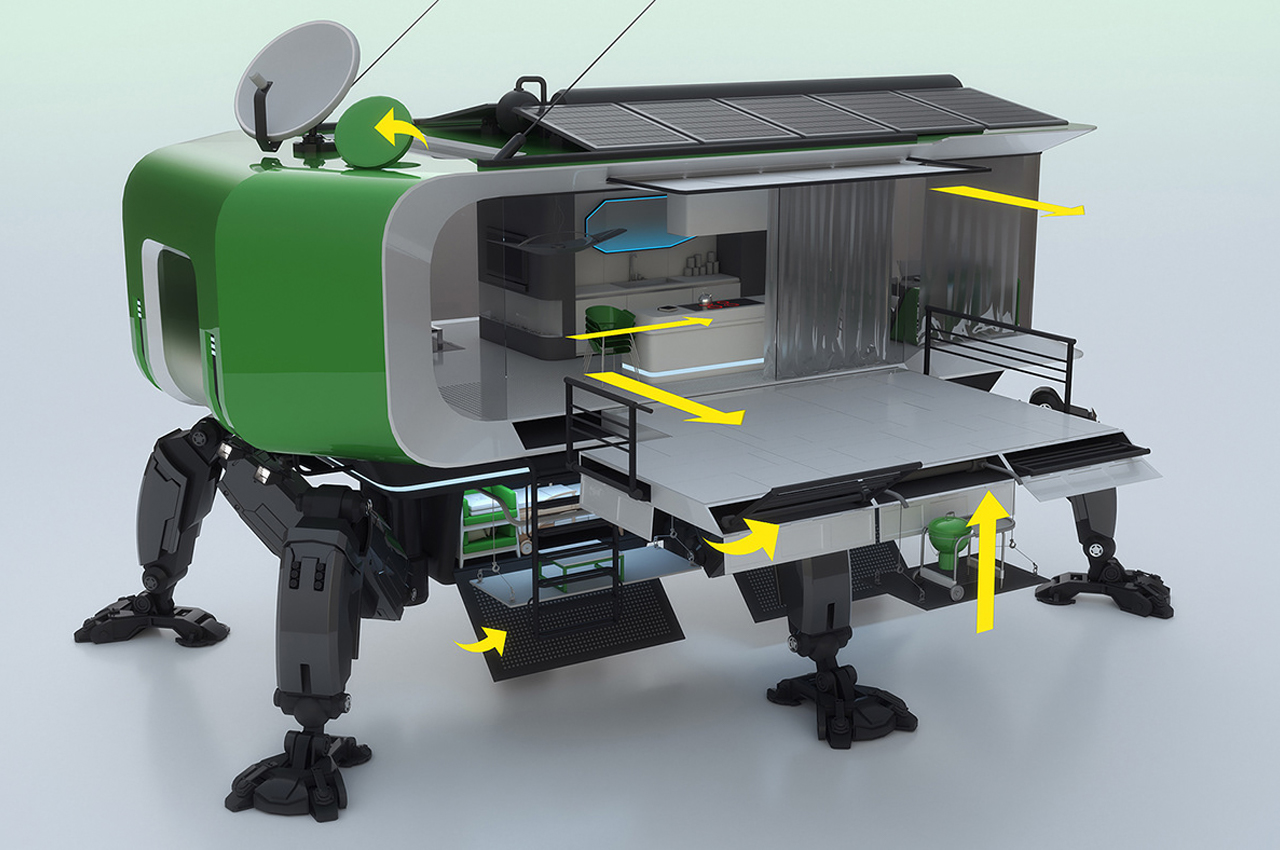The image showcases a highly detailed model of a futuristic, mobile house elevated on large black mechanical legs. The house features a green exterior with light green paint, a black-railed deck area in front, and is equipped with both green and gray satellite dishes as well as solar panels on the roof. Entry to the house appears to require climbing a vertical ladder of about four or five steps. Inside, the kitchen area includes a white island and counters, a green chair, and a stack of cans in the right corner. Additional features inside include arrows pointing to the stove and other parts of the house, as well as small gray curtains on the windows. The overall design is surprising and exceptional, resembling a modern trailer home but with an elevated and innovative twist.